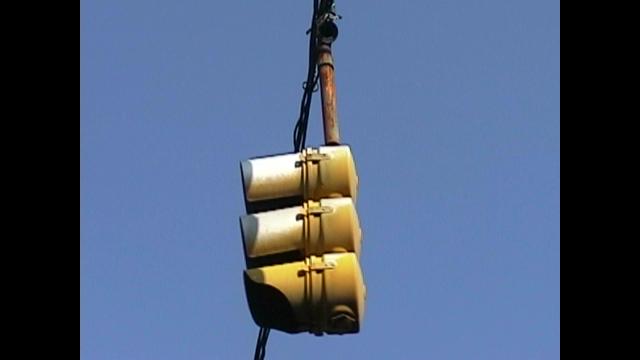In the image, a large metal pipe extends down from the top, framed by black borders on both sides. Against a clear blue sky, the pipe is intricately wrapped with several cords of varying thicknesses. These cords are securely holding and lifting three sizable, drum-shaped containers. Each container has a black bottom and a light brown body. The containers appear to be in the process of being hoisted up, with the cords meticulously wrapped around them, towards the long rod that continues upward and out of the frame.